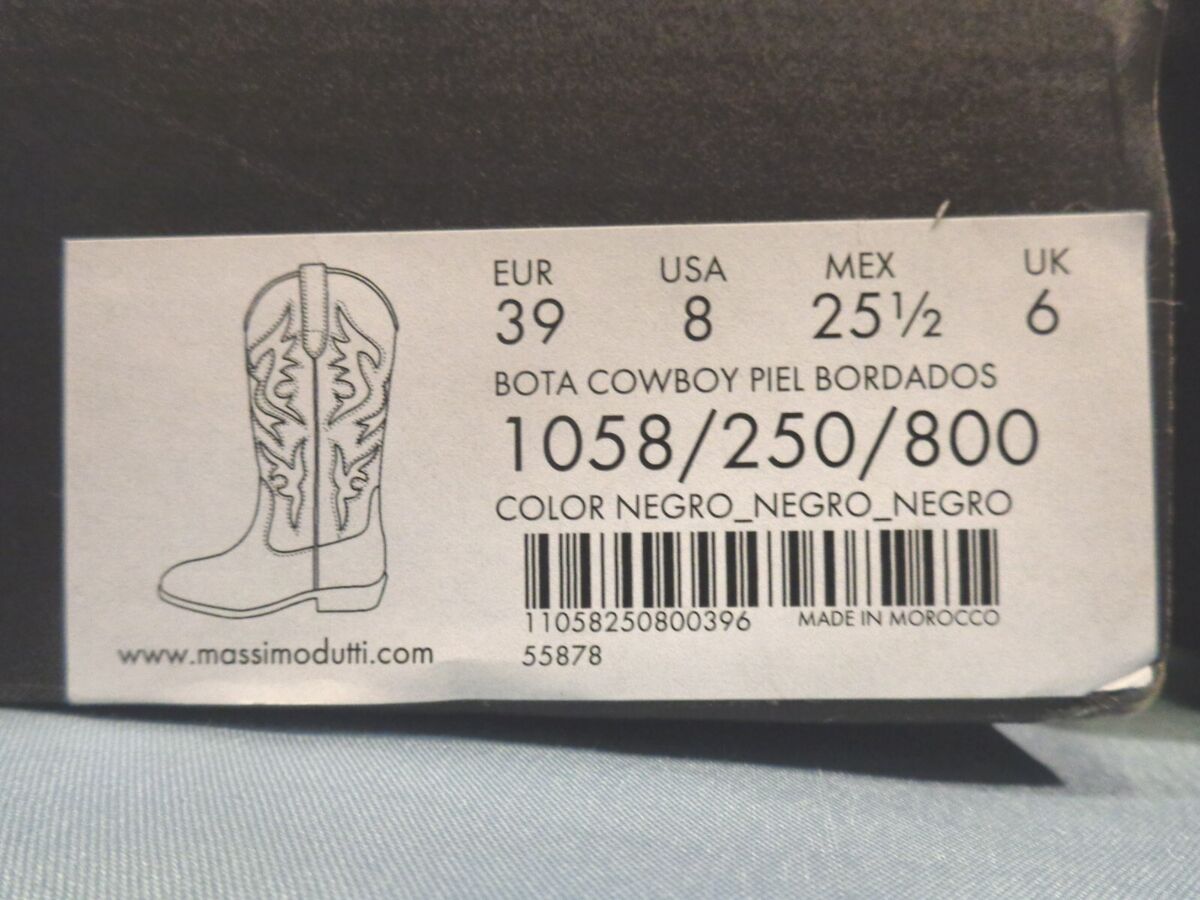The image features a beige label affixed to a brown wooden surface, likely a shoe box. The label, written in dark brown text, provides detailed information about a product—black cowboy boots from the brand Massimo Dutti. The label specifies the sizes: EUR 39, USA 8, Mexican 25.5, and UK 6. It prominently states "Bota Cowboy Piel Bordados," with the color described as "Negro-Negro-Negro." Additionally, there is a barcode and the model number "1058-250-800." Below a black outline drawing of the boot, the website "www.massimodutti.com" is printed, indicating the brand's official site. The detailed design and multilingual information hint at the boots' international market availability and the emphasis on their black color in Spanish.